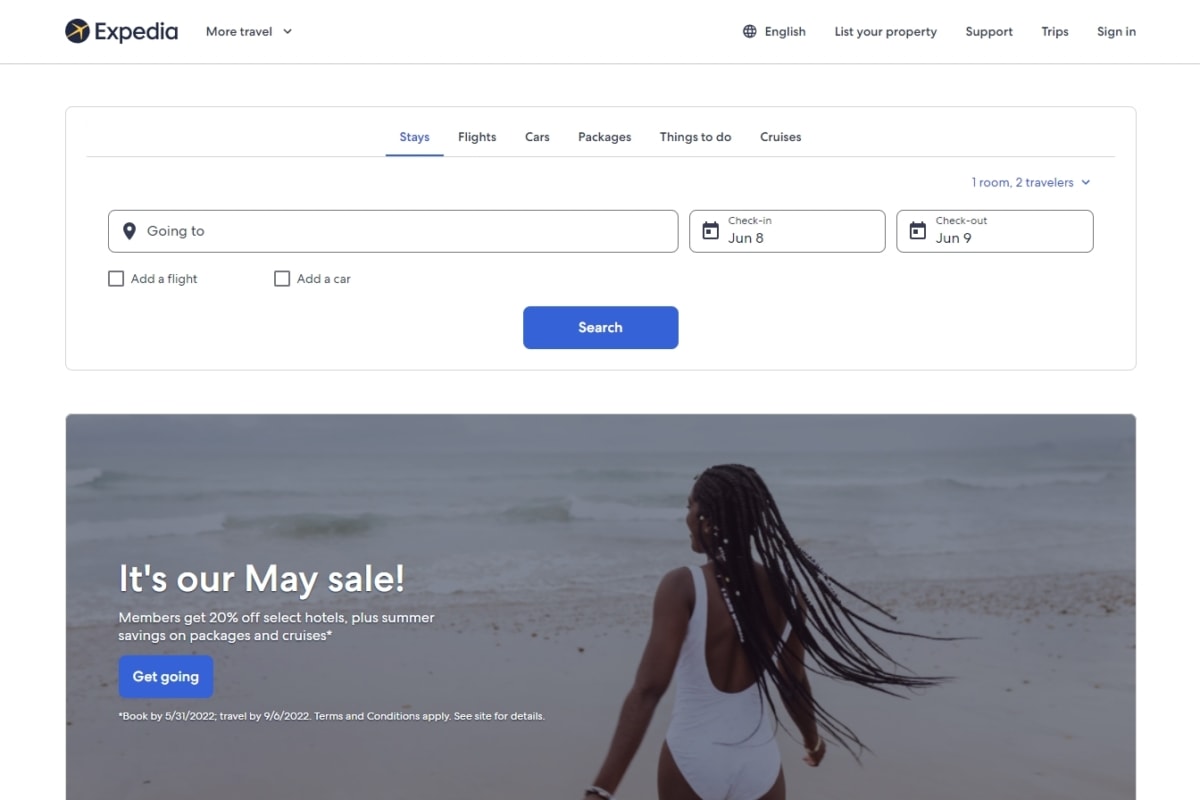The image depicts an Expedia webpage featuring its name and logo positioned in the top left corner. Adjacent to this is a "More Travel" drop-down menu. To the right, there's an option to change the website's language, currently set to English. Additional links include options to list a property, access support, view trips, and sign in to the platform. 

Dominating the upper section of the webpage is a comprehensive search bar. Users can specify their search criteria by selecting categories such as stays, flights, cars, packages, things to do, and cruises. The current selection is "stays." Users can further input their travel destination, flight details, car preferences, check-in, and check-out dates. Beneath this section, a prominent blue "Search" button allows users to execute their query.

The lower half of the image features a vibrant photo of a Black woman in a bathing suit walking towards the sea across a sandy beach. To the left of this image, in white text, is an announcement for Expedia's May sale, stating, "Members get 20% off selected hotels plus summer savings on packages and cruises." Below this text, another blue button labeled "Get Going" invites users to take advantage of these offers.